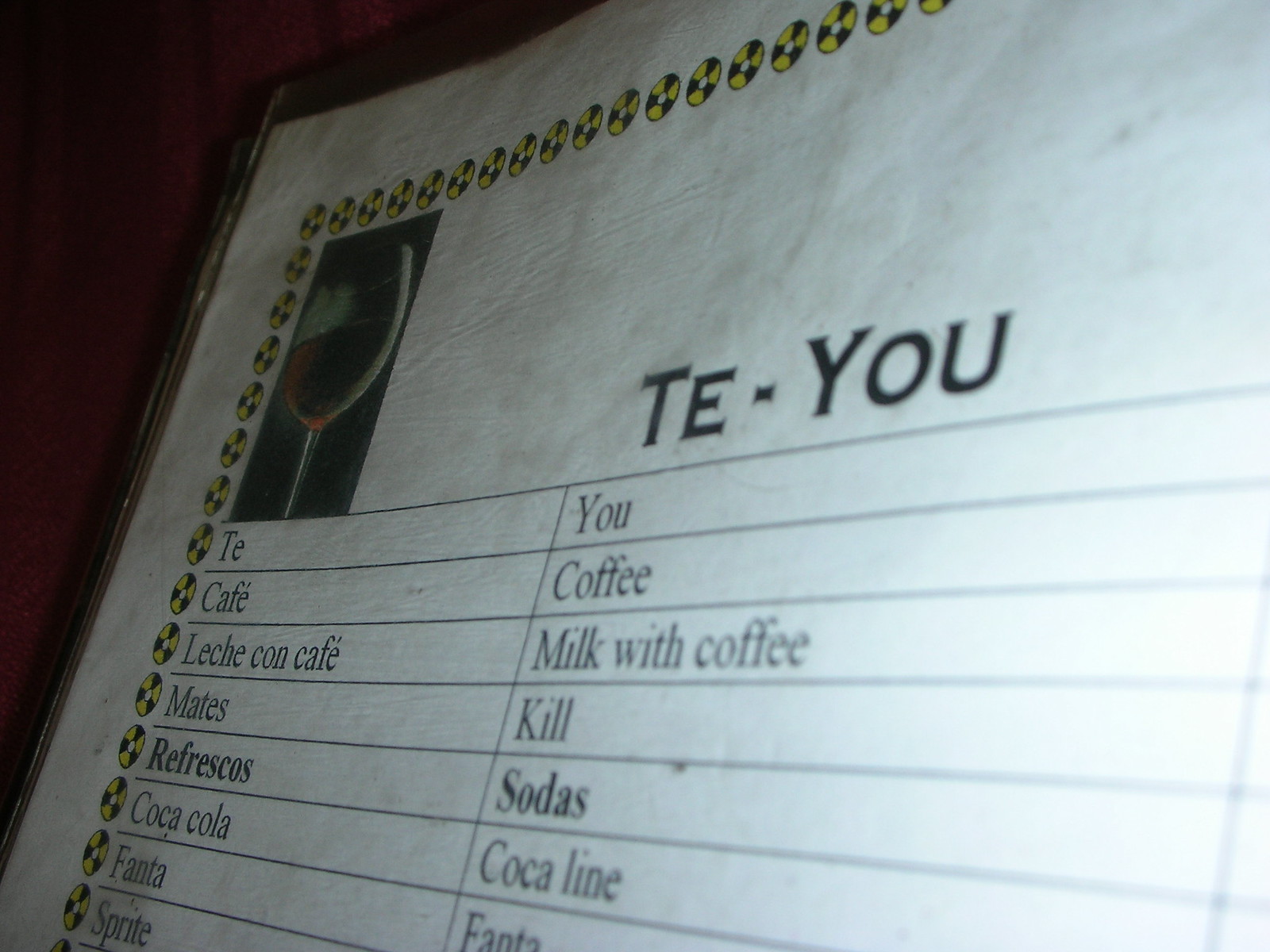The image depicts a laminated menu with a circular yellow and black hazard-like border. At the center top of the menu, in bold letters, reads "TUTE-YOU," followed by bracketed texts resembling spreadsheet format. On the top left of the menu is a photograph of a wine glass filled halfway with red wine. To the left side, from top to bottom, it lists items in another language: "TE CAFE LECHE CON CAFE MATES FRESCOS COCA-COLA FANTA SPRITE." The corresponding English translations on the right side read: "YOU COFFEE MILK WITH COFFEE KILL SODAS COCA-LINE FANTA," although part of the text at the bottom is cropped out. A light source reflects off the laminated surface to the right, and the background reveals a dark red (maroon) wall predominantly visible at the top corners of the image.